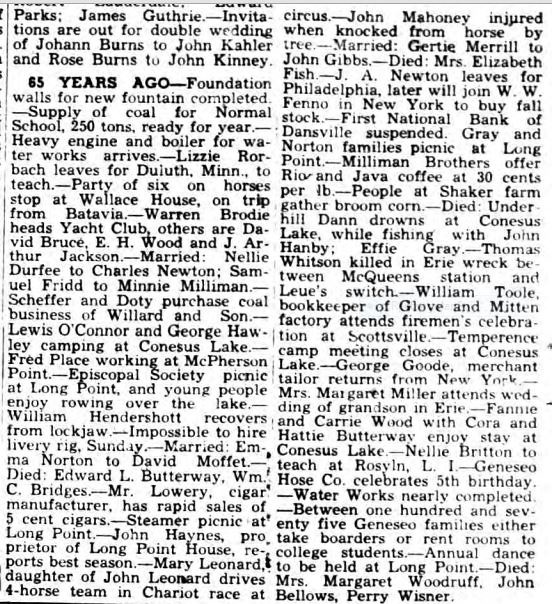The image depicts a slightly faded, old-school newspaper clipping dominated by two extensive columns of black, bold text on a white background. This newspaper text appears to be a screenshot or a scan, and the text is cropped at the edges, suggesting it is part of a larger article. The first column starts at the top left with an announcement of a double wedding: "Invitations are out for a double wedding of Johan Burns to John Koehler and Rose Burns to John Kinney." This is followed by historical notes: "Sixty-five years ago, foundation walls for a new fountain were completed, and a supply of 250 tons of coal for the normal school was prepared for the year. A heavy engine and boiler for the waterworks also arrived." The second column, which begins at the upper right, includes various news items such as "John Mahoney injured when knocked from horse by tree" and ends with local events and obituaries, mentioning "Annual dance to be held at Long Point" and "died Mrs. Margaret Woodruff, John Bellows, Perry Wisner." The overall presentation and slightly fuzzy, faded print indicate the age and authenticity of the newspaper clipping.